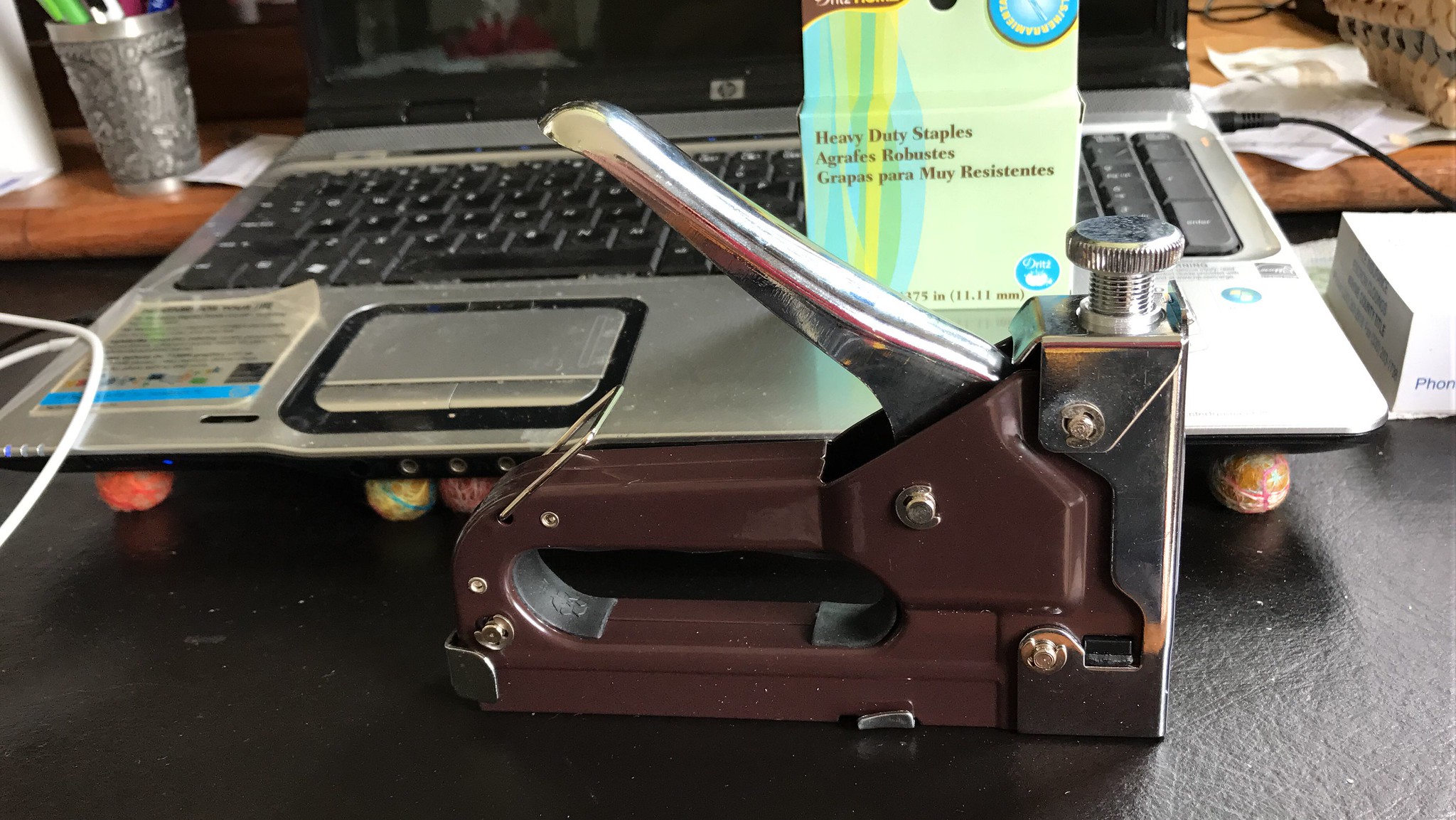This indoor color photograph showcases a desk scene centered around an HP laptop with a silver-gray body and black keys. The laptop is propped up by four bouncy balls: red and orange at the corners and yellow and red in the middle, providing an unusual makeshift stand. A box of "heavy duty staples," unopened and adorned with green, blue, and yellow stripes alongside multilingual text, rests on the laptop's keyboard. In front of the laptop, prominently displayed on the desk's black surface, is an old-fashioned industrial-style stapler with a dark brown or deep maroon body and metallic silver parts. The scene is further detailed by the presence of a shelving unit behind the laptop, holding paper and a cup filled with pens. A power cord connects to the laptop, contributing to the workspace's organized yet functional aesthetic.